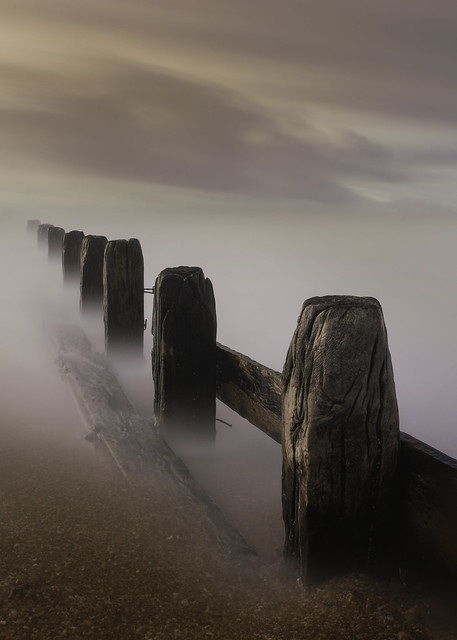This photograph is shrouded in a dense haze and fog, rendering most of the background a whitish-grey blur. The main feature in the image is an old and weathered wooden railing that extends perpendicularly to the left, fading into the fog. The railing is composed of thick, vertical wooden pillars or stumps, which are two to three feet tall and marked by time-worn ridges and some protruding metal pieces. Between these vertical stumps, several horizontal wooden boards are present, though some are missing, accentuating the railing's aged appearance. The ground at the bottom is covered in a rocky or sandy brown material, adding to the rugged, possibly desert-like, setting. The fog is so dense that it almost merges with the clouds, giving an illusion of the railing being above the clouds or a city.